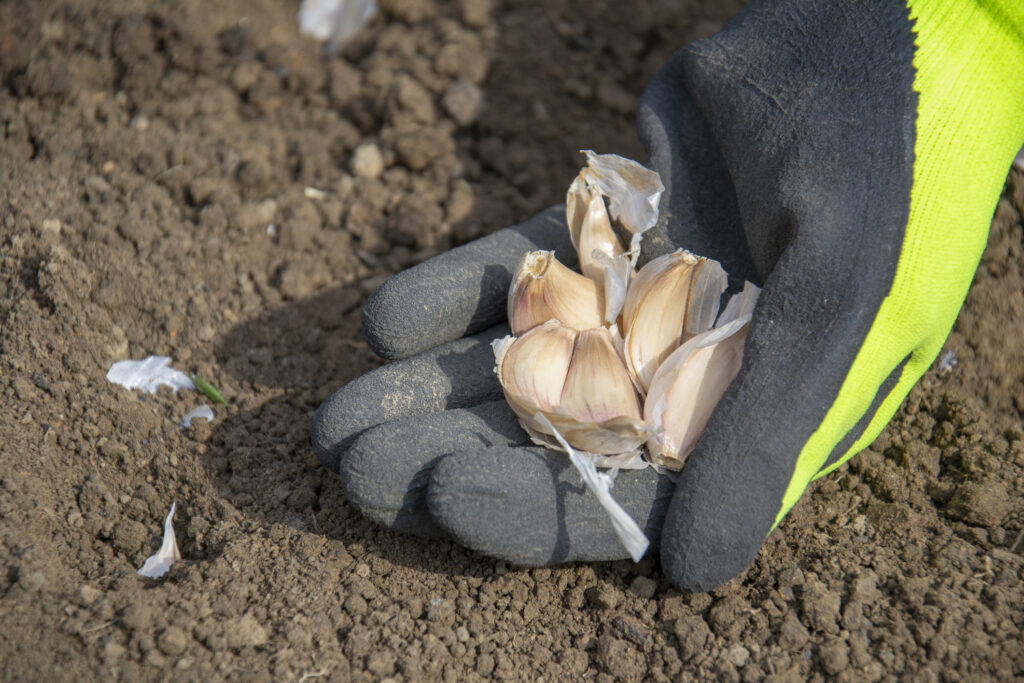The image depicts a left hand wearing a gardening glove, resting on a patch of dry, clumpy brown dirt. The glove is neon yellow-green on the back and gray on the palm, which appears textured. The gloved hand, positioned towards the right side of the image and oriented with the fingers pointing to the lower left corner, is holding six garlic cloves. Three cloves near the fingertips are clustered together, while the other three near the base are slightly separated but still close to the group. Scattered across the dirt are small pieces of garlic skin, adding to the organic and earthy setting.